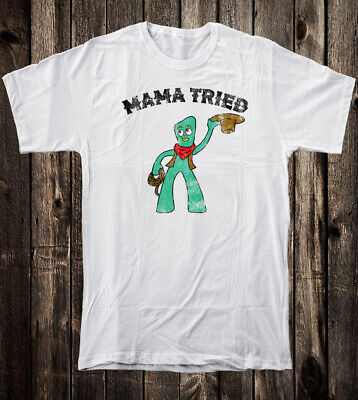This photograph shows a white, short-sleeved crew neck T-shirt spread out on a weathered, rustic wooden table with visible knot holes and a distressed brown finish. The T-shirt features an illustration of Gumby, the iconic green clay character. Gumby is depicted wearing a red bandana around his neck and holding a cowboy hat upside down in his left hand, as if doffing it. In his right hand, near his hip, he's clutching a coiled rope. Above Gumby's head, a curved line of text in black, capital letters reads "MAMA TRIED," adding a humorous touch to the cowboy-themed design. The overall scene conveys a nostalgic, Americana feel.